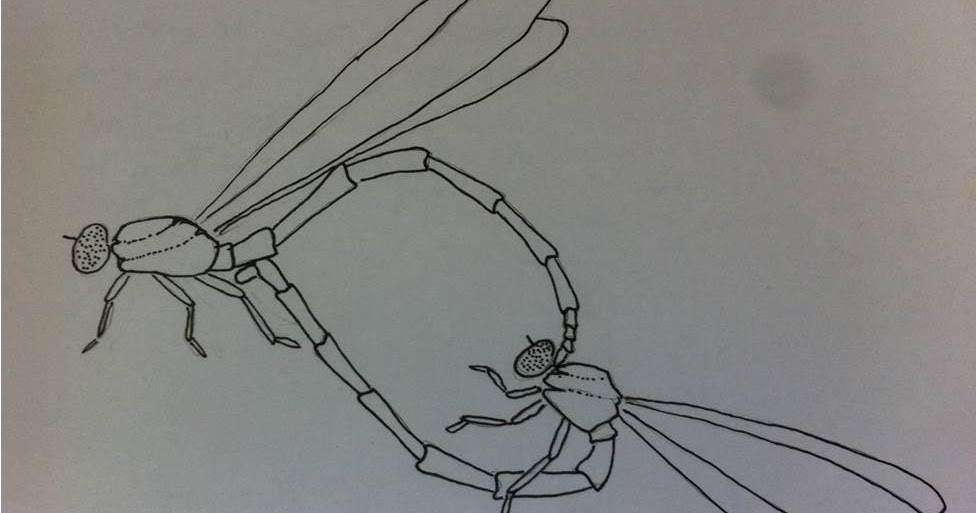In this detailed line drawing on a gray background, two dragonfly-like insects are intricately entangled by their tails, creating a dynamic scene that evokes both conflict and connection. Each insect's tail is long and sectionalized, with at least six or seven distinct segments ending in a pointed tip. The insects exhibit slender wings and typical insect heads, characterized by small swivels on their necks for mobility, along with distinctly larger and thicker abdomens. Both insects have six legs, arranged symmetrically with three on each side. The drawing captures speckled eyes and dotted body markings, enhancing the intricate detail of the sketch. There is an additional dark gray circular marking, somewhat resembling a skull, in the top right corner, adding an enigmatic element to the composition. Despite its amateurish appearance, the sketch imbues a sense of depth and possibly symbolic meaning as it depicts the interaction or struggle of these two insects.